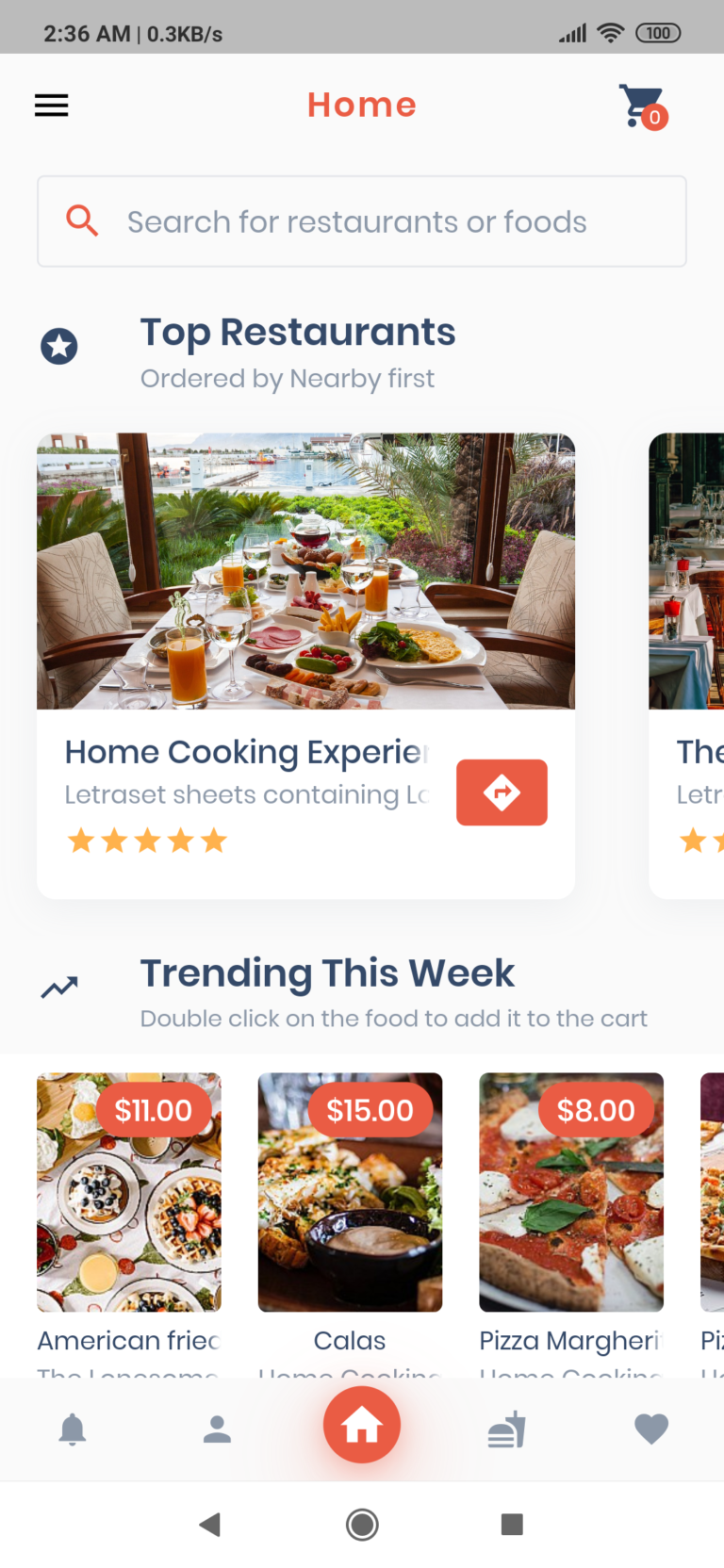This screenshot showcases a menu interface from a food delivery or restaurant app. At the top, users can see a "Home" button next to a shopping cart icon featuring a solid yellow or orange circle with the number zero inside, indicating no items in the cart. The menu highlights "Top Restaurants Ordered By Nearby" and provides a brief description of the "Home Cooking Experience," rated with five stars.

Below this, there's an option to scroll through images and a search bar prominently displayed for easy navigation. The section titled "Trending This Week" lists popular menu items with corresponding details:

1. **American Fried Chicken** - Priced at $11, users can double-click to add this item to their order.
2. **Calas** - A soup dish, priced at $15.
3. **Pizza** - Offered at $8.

Additional icons at the bottom feature an orange circle with a white house, an alarm, a person, and symbols for food and drink, as well as a "Favorites" section. Users can easily scroll forward and backward through the colorful and vibrant pictures of menu items.